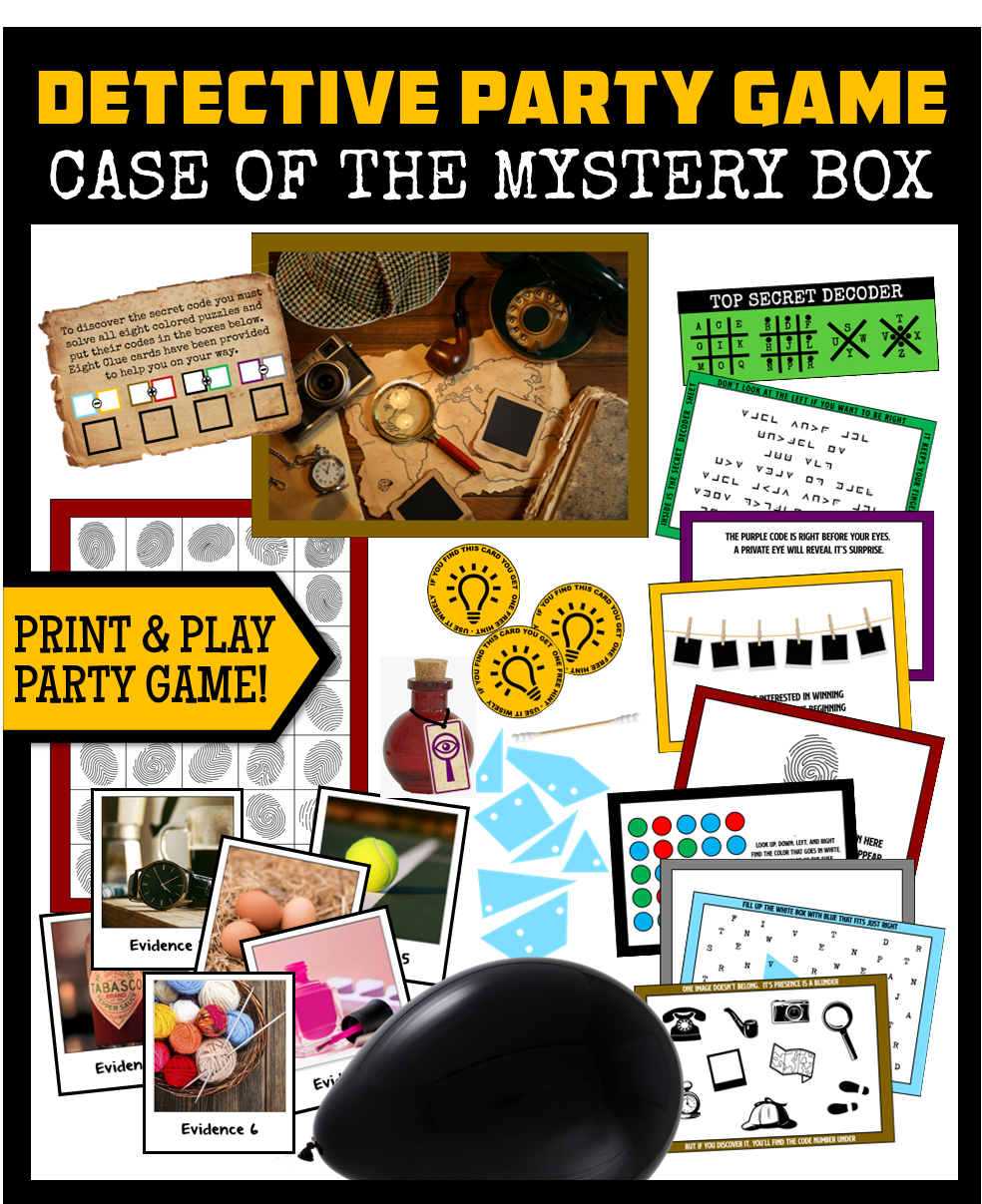This image is a detailed advertisement for a detective-themed party game. At the top of the image, in bold, thick, yellow capital letters, it says "DETECTIVE PARTY GAME," set against a black header. Below, in squiggly white capital letters, the text reads "CASE OF THE MYSTERY BOX." The background just below this is also black, providing a striking contrast. In the middle of the image, there is a variety of items associated with the game. On the left side, there is a series of six Polaroid-style photos labeled "Evidence," featuring images of a watch, eggs, a tennis ball, nail polish, a basket of yarn, and Tabasco sauce. In the foreground at the bottom center, there is a black balloon lying on its side.

To the right of the evidence photos, there is a stack of postcard-like images showcasing elements of the mystery, such as cipher keys and grids, which appear to be part of the game's puzzles. There are additional postcard-style photographs that seem to be hanging and drying, along with images of thumbprints and more puzzles. At the top, there is a "Top Secret Decoder," presented in a rectangular box with tic-tac-toe-like grids and other cipher elements, some bordered in green.

On the left side of the image, there is a prominently displayed thick, yellow arrow with a black border pointing inward. Inside the arrow, in all capital yellow letters, it reads "PRINT AND PLAY PARTY GAME," indicating the game's format.